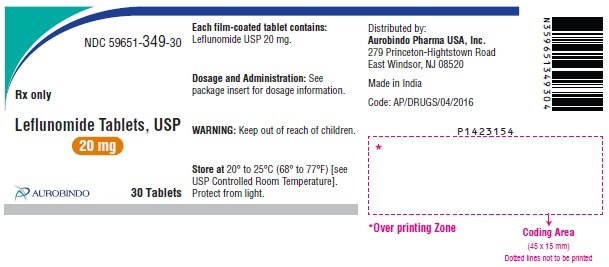The image features a prescription label for Leflunomide tablets, USP 20 milligrams, from Aurobindo Pharma USA Inc. In the upper right-hand corner, there is a vertically-oriented barcode with the numerical sequence displayed sideways. Adjacent to this barcode is a white box outlined with pink dotted lines containing a pink star that reads "Overprinting Zone." Just below this, a pink arrow points downward, indicating a "Coding Area, 45 by 15 millimeters," and it is noted that the dotted lines should not be printed. 

In the center of the label, the text specifies that the prescription is for 30 film-coated tablets, each containing 20 milligrams of Leflunomide USP. It advises users to "See package insert for dosage information" and includes a warning to "Keep out of reach of children." Storage instructions indicate that the medication should be kept at 20 to 25 degrees Celsius, following USP controlled room temperature guidelines, and should be protected from light.

The bottom left corner of the label displays the name of the distributing company, "Aurobindo Pharma USA Inc," located in East Windsor, New Jersey. The product is manufactured in India.